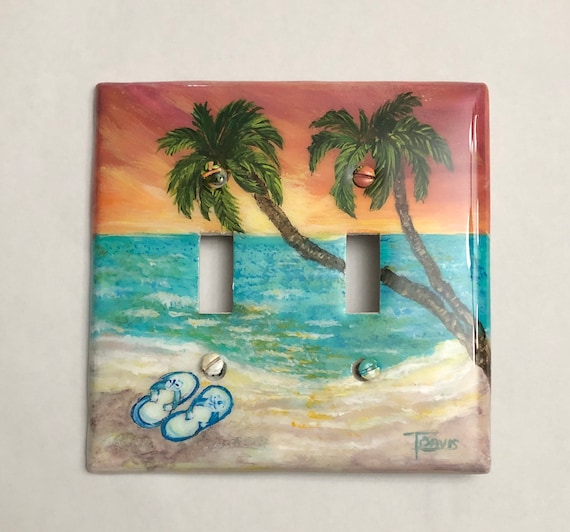The image is a detailed color photograph of a painted wall outlet cover designed for two adjacent light switches. The cover is adorned with a vivid tropical beach scene. Dominating the design are two palm trees emerging from the bottom right corner and leaning diagonally towards each other. The palms extend across the open switch holes, creating a cohesive flow. At the beach scene's base, two blue sandals lie as if casually discarded, adding to the relaxed atmosphere. The serene blue water extends in the background, leading up to an orange and red sunset sky that gradually blends into yellow hues. The outlet cover's surface is interrupted by four flathead screws that are integrated into the painting. The artwork is signed in the bottom right corner with what appears to be the name "F O A V I S." The cover is set against a plain white background, emphasizing the artistic detail and tropical essence of the painted scene.